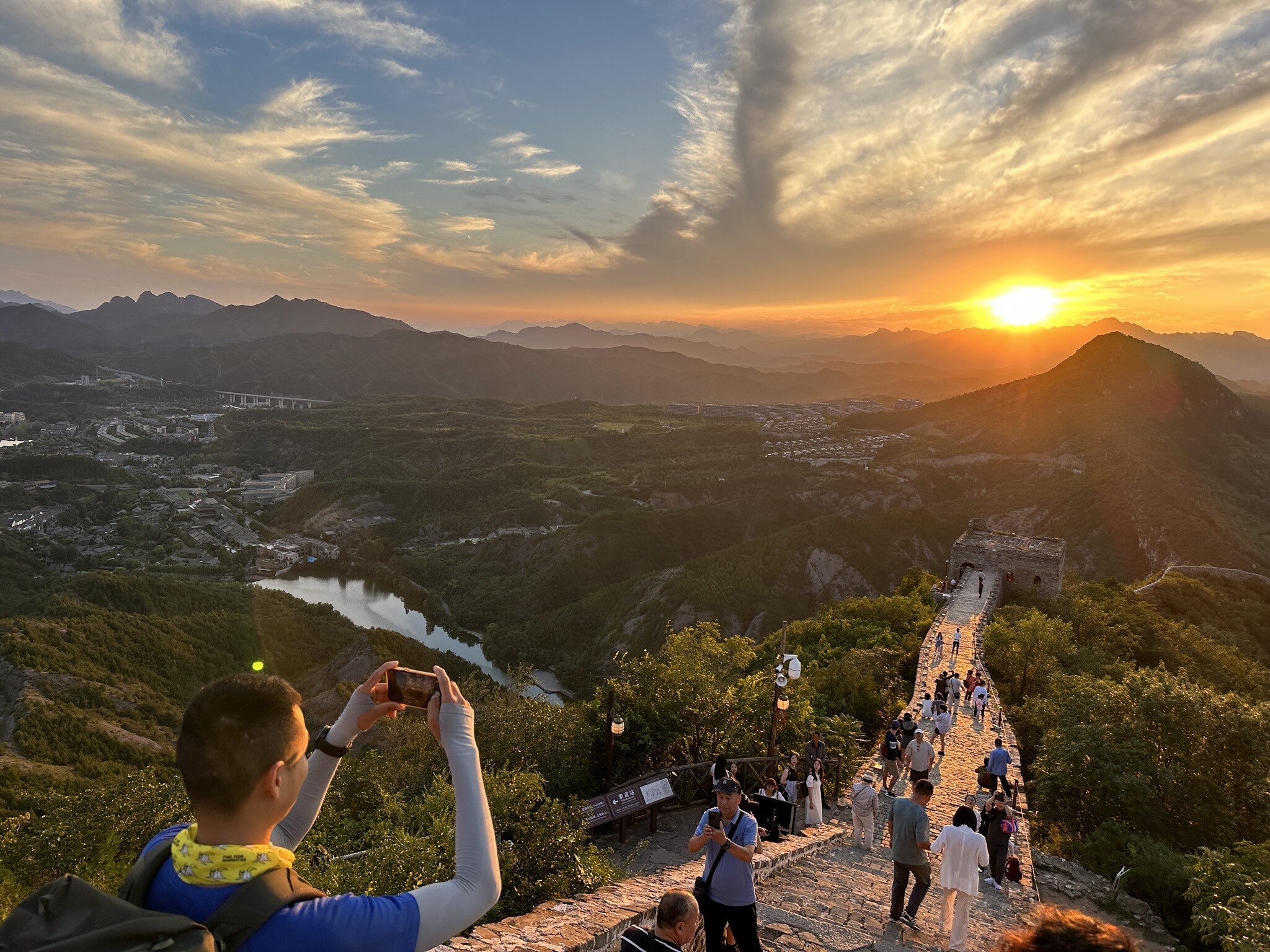In this detailed outdoor photograph at the Great Wall of China, a person wearing a blue shirt and carrying a backpack is prominently featured in the bottom left corner, holding up a cell phone to capture the scene. They stand at the edge of a stone pathway that stretches from the foreground to the background, highlighting the iconic architecture of the Great Wall as it extends across the mountainous terrain. The wall is dotted with dozens of tourists exploring this historic site. Above the right side, the sun is seen rising over the distant mountains, casting an orange glow onto the scene. The sky transitions from a dusky yellow near the horizon to a deeper blue towards the top, interspersed with a decent cloud cover throughout. To the left, a river or lake can be seen, with a town situated on its far side, and another town lies further out near the center right close to the mountains. The landscape is lush with trees surrounding the Great Wall on both the left and right, enhancing the natural beauty of the setting.